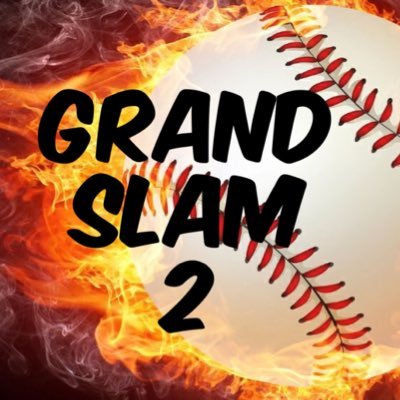The image is a vivid, square graphic depicting a dramatic baseball scene filled with dynamic, colorful elements. It features a large white baseball with prominent red stitching taking up the entire right side of the image. The ball appears to be flying through the air, trailing intense flames in bright yellow, orange, red, and gold hues that span from the middle left to the center of the composition. The upper left and bottom right corners of the background are dark brown with swirling white patterns, while the rest of the background has a dark red or maroon tone, adding depth and contrast to the fiery spectacle. Superimposed boldly in the center, in large black capital letters, the text reads "Grand Slam 2" arranged on three lines. The dramatic imagery, combined with the striking typography, suggests the image could be an advertisement for something related to baseball, possibly a video game or event titled "Grand Slam 2."